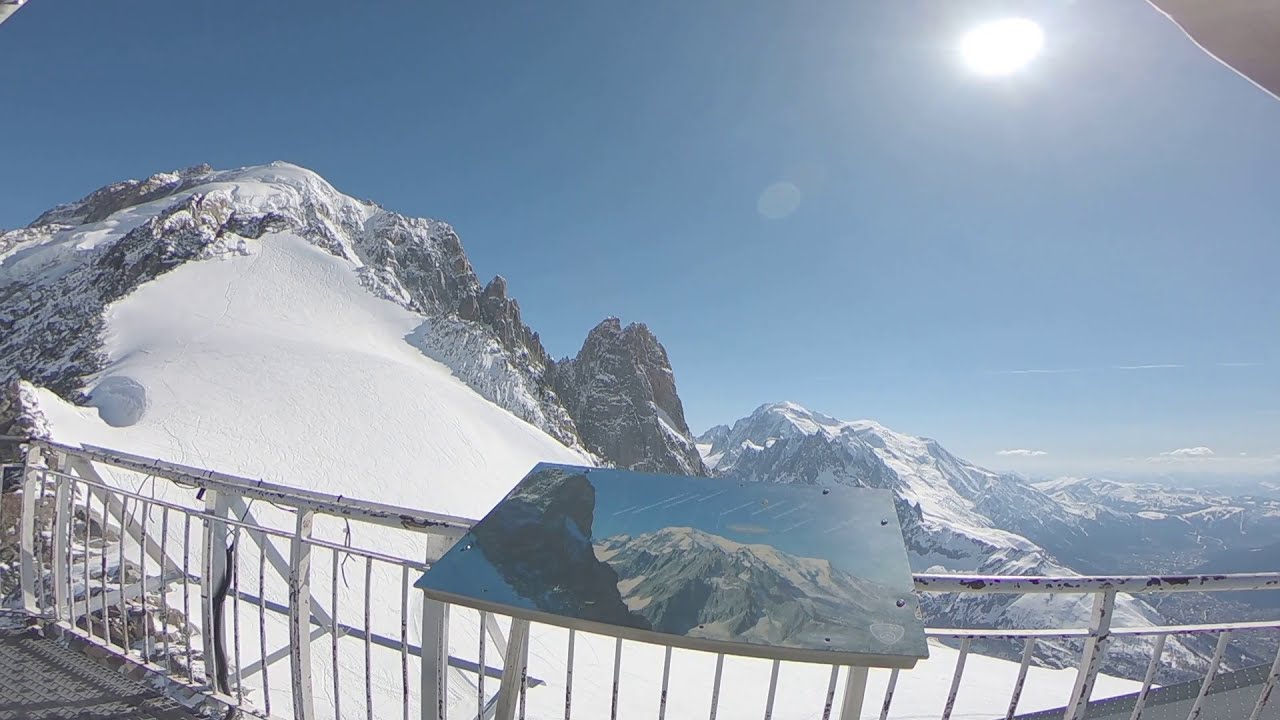The image is a detailed photograph taken outdoors, showcasing a vast, snowy mountain range. The vantage point is from a balcony or ledge, likely made of gray steel, featuring a white railing and a public walkway for better viewing. In the foreground, there's a large plaque or picture mounted on the railing, depicting the same snowy mountains seen in the background. This plaque might include some text or diagrams about the mountains. The mountains themselves stretch across the image, with the highest peak fitting into the upper left corner. The sky above is mostly clear with a few thin white clouds near the horizon, and the bright sun is prominently positioned in the top right corner. The overall scene is well-lit with natural daylight, emphasizing the smooth, expansive white snow covering the rugged mountain peaks.